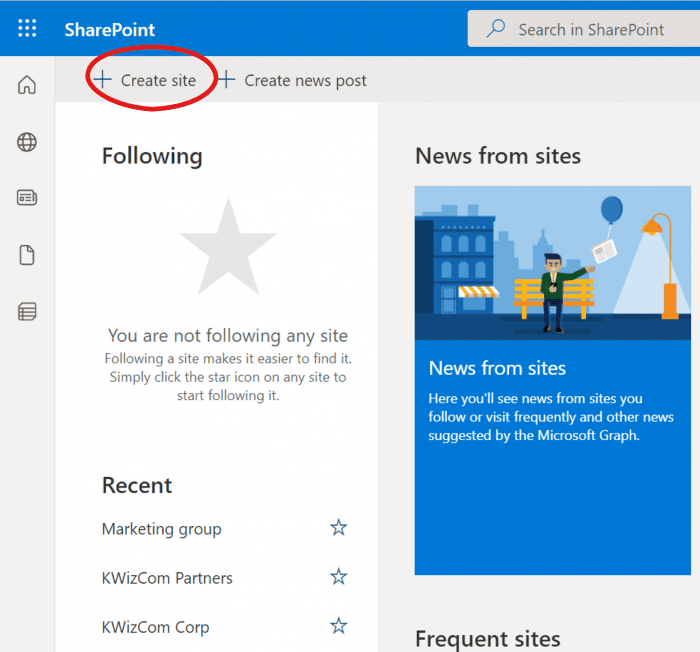The screenshot showcases a SharePoint website with the left and bottom edges cut off, rendering the right side of the page out of view. At the top of the page is a distinct blue band featuring a 3x3 grid icon composed of nine squares or dots, and the word "SharePoint" written in white text. Central to the interface is a prominent white search bar labeled "Search in SharePoint".

A red circle, added via a photo editor, highlights the "Create site" option situated at the top left corner. This option is represented by a blue plus symbol and the text "Create site" in black. Adjacent to "Create site", and also circled, is the "Create news post" option. 

Running down the left side of the screen is a navigation bar with various icons: a house, a globe, a sheet of paper with lines, a folded sheet of paper, and a rolled paper scroll. Below the "Create site" option, there is a section labeled "Following" that features a gray star icon and a text that states, "You are not following any site. Following a site makes it easier to find it. Simply click the star icon on any site to start following it."

Three listed sites—Marketing group, KWIZ.com partners, and KWIZ.com corp—appear below this message, each accompanied by an outlined star icon on the right, denoting the option to follow these sites.